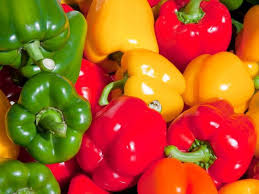This vibrant photograph showcases a variety of glossy bell peppers in green, red, yellow, and even a hint of orange. The peppers, numbering over twenty, are piled and scattered across the image, creating a colorful and enticing display. On the left side, the dark green bell peppers with lighter streaks are predominantly gathered, while the bottom middle features the bright red peppers. Near the bottom right are the lighter yellow peppers, interspersed with orange hues, contributing to the vivid contrast. At the top, a mixture of yellow, red, and green bell peppers are stacked, their thick green stems prominent. Each pepper has noticeable indents running down its sides and reflects a white light, enhancing their glossy appearance. The overall composition resembles a well-organized chaos, similar to a display one might find at a farmer's market or online store, drawing attention to the fresh, appealing produce.